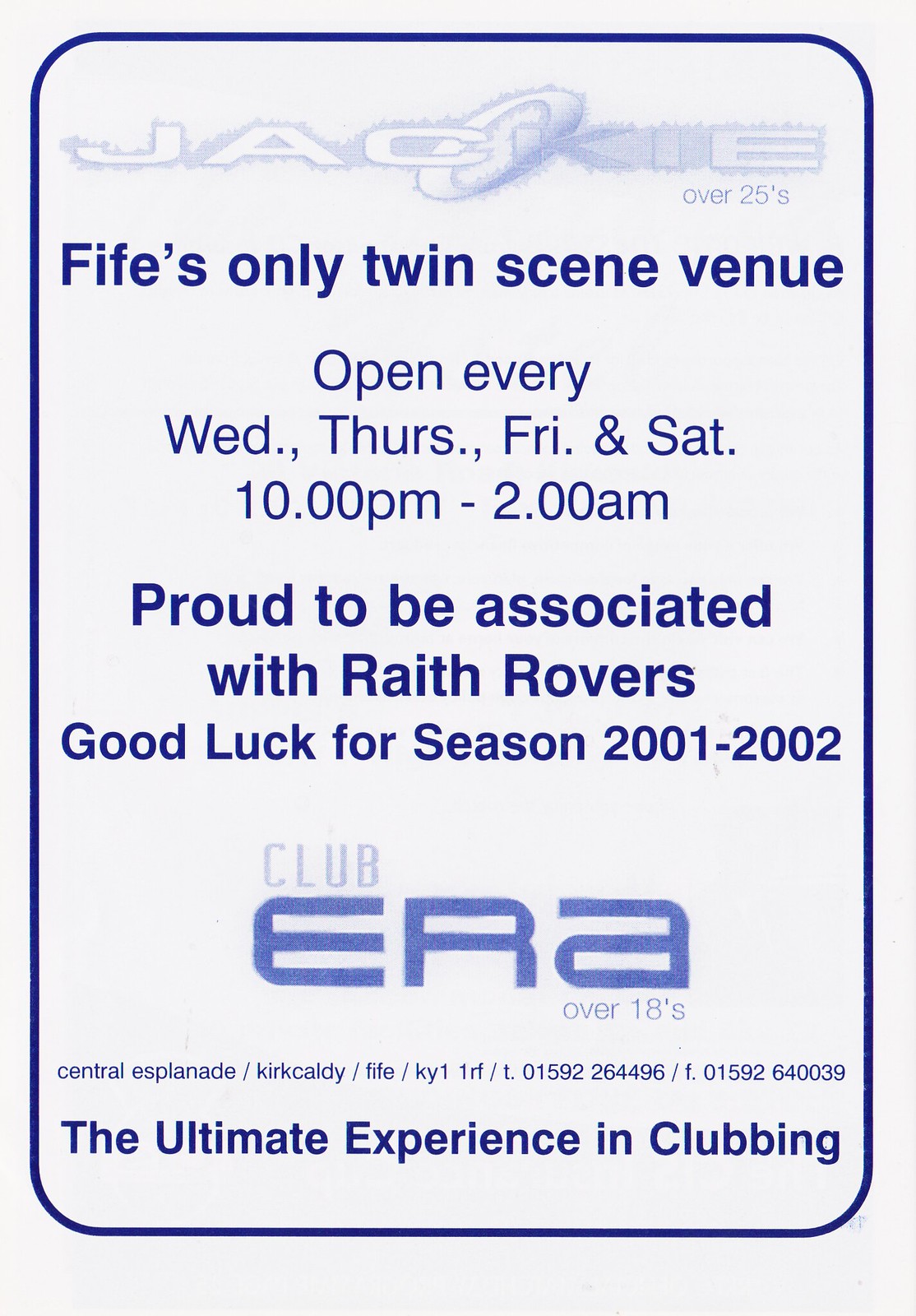This image depicts a promotional poster primarily featuring a light grey background and enclosed in a blue-bordered rectangle with rounded corners. The text, all written in blue, begins at the top with "Jackie over 25s," the word "Jackie" adorned with an oval shape on its tilt. Below, it highlights "Fife's only twin scene venue, open every Wednesday, Thursday, Friday, and Saturday from 10:00 p.m. to 2:00 a.m." The club proudly associates with Raith Rovers and wishes good luck for the season 2001-2002. Further details include a logo with "Club Era over 18s," followed by the location "Central Esplanade, Kirkcaldy, Fife, KY1 1RF," and contact numbers "telephone 01592-264496" and "fax 01592-640039." The tagline at the bottom boldly states, "The ultimate experience in clubbing."